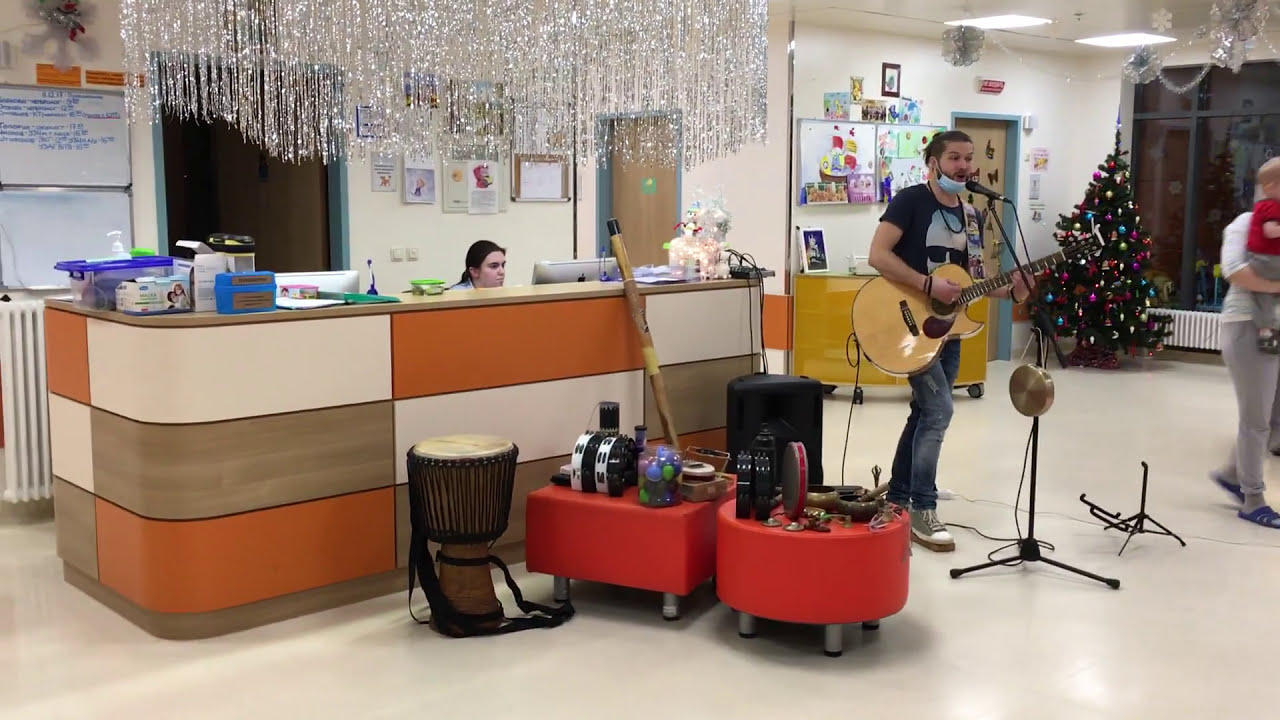In this detailed photograph, a man stands as the focal point, passionately playing an acoustic guitar in what appears to be a nurse's station or an office-like area, likely within a hospital. He is dressed casually in a black t-shirt with an insignia, blue jeans, and gray sneakers. His light blue COVID mask is pulled down below his chin, revealing his facial hair and ponytail. The man, engrossed in his performance, sings into a microphone while surrounded by his complete set of musical equipment.

Adjacent to him are orange stools, cluttered with various instruments including tambourines, bells, singing bowls, and cymbals. Behind him, there is a standing drum. This festive scene is accentuated by a Christmas tree positioned in the right corner and glittery, icicle-like tinsel draped from the ceiling above a desk. The desk, appearing to be a receptionist or nurse's station, has a dark-haired nurse sitting behind it, focused on a computer amid typical hospital items like boxes of wipes and hand sanitizer.

Additionally, two tables—one round and one square—stand to the musician’s right, holding game-oriented objects. The setting hints at an event or concert held for Christmas, evidenced by the festive decorations and the faintly industrial or office-like backdrop. This celebratory atmosphere is further marked by a person holding a child, seen near the edge of the frame, adding to the communal and joyous spirit of the occasion.